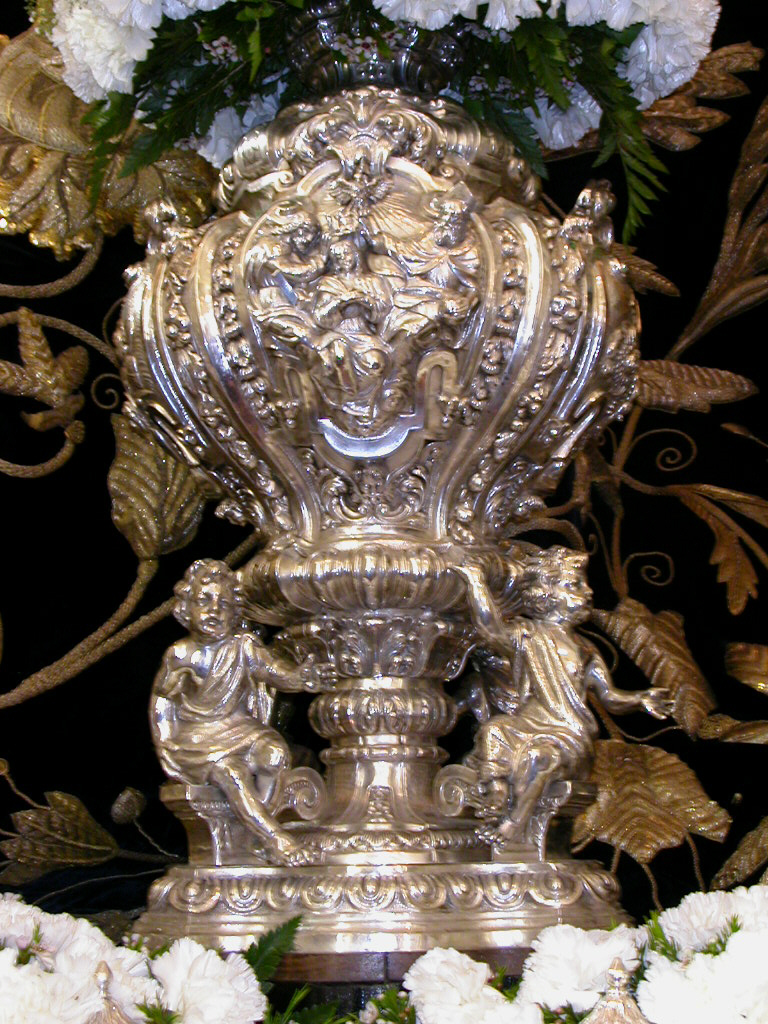The photograph captures a highly ornate and reflective vase, predominantly featuring a silver and bronze color palette. The vase presents a rich array of decorative elements, starting from its rounded base which supports the expansive, intricate design. At the narrow neck just above the base, two small, cherubic figures with curled hair and robed garments are seated on opposite sides, each holding the base with outstretched arms. The vase's design flourishes with elaborate patterns of flowers, beams, and curves that ascend towards the top.

Distinctly bulbous in the middle, the vase tapers elegantly towards the top. Here, an angelic figure appears to look down amidst an intricate arrangement of emblems and designs. The vase is crowned with a display of large white flowers accompanied by green leaves, further enhancing its decorative appeal. Additionally, similar white flowers and green leaves are scattered toward the bottom of the image, contributing to the cohesive floral theme. The background of the image is adorned with ornamental wallflowers and shiny bronze leaves, complementing the vase's opulent and sacred aesthetic.